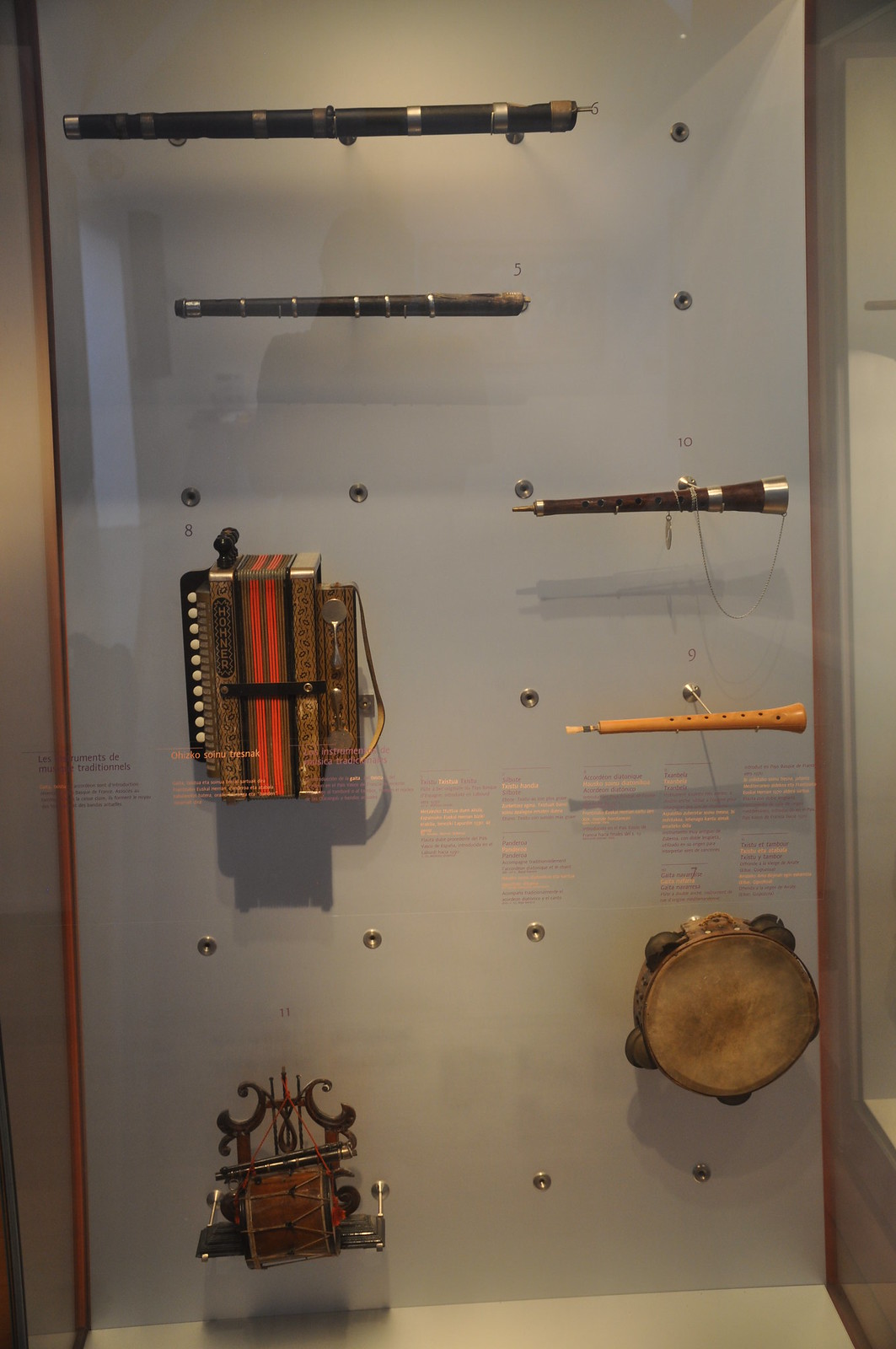The image depicts a rectangular, glass-covered display cabinet showcasing various historical musical instruments. At the top of the display, two black flutes are prominently mounted. Below them, a pointed brown flute and, further down, a light wooden tapered flute are displayed. Centrally, the cabinet features what appears to be a small accordion-like box, possibly an antique accordion. To the right, there's a tambourine, and to the left, there are two small drums, with one featuring leather and metal arms for rhythm-making. The instruments are attached to the white back of the cabinet with silver rings, and descriptive labels are affixed to both the items and the outside of the glass, although the text is not legible.